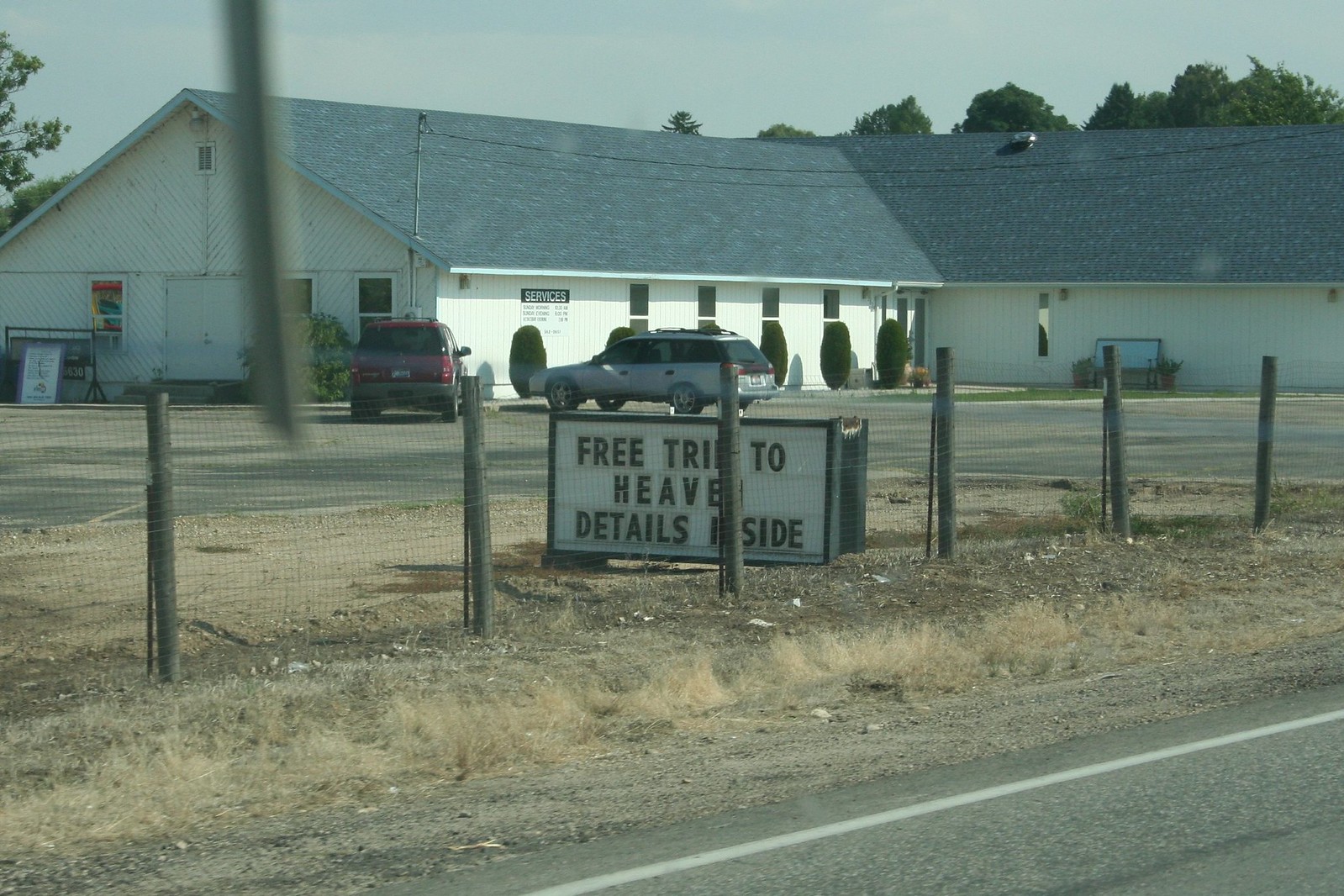In this outdoor scene, we see a photograph likely taken from a moving vehicle that captures an L-shaped, off-white church with a grayish roof and long vertical windows. Prominently displayed in front of the building is a white sign with black letters that partially obscures the text, likely reading, "Free trip to heaven, details inside." The sign is accompanied by a series of wooden posts and fencing that could be chicken wire. In front of the church are two parked cars on a grayish-brown road that includes a white stripe marking the edge of the lane. Surrounding the parking lot is a stretch of dead grass. The entrance to the church, featuring two doors, is located on the left-hand side of the building, with a bench nearby for waiting visitors. An air vent is visible on the roof to the right side. The background of the photograph shows a light blue sky without clouds, with some trees peeking out from behind the church.